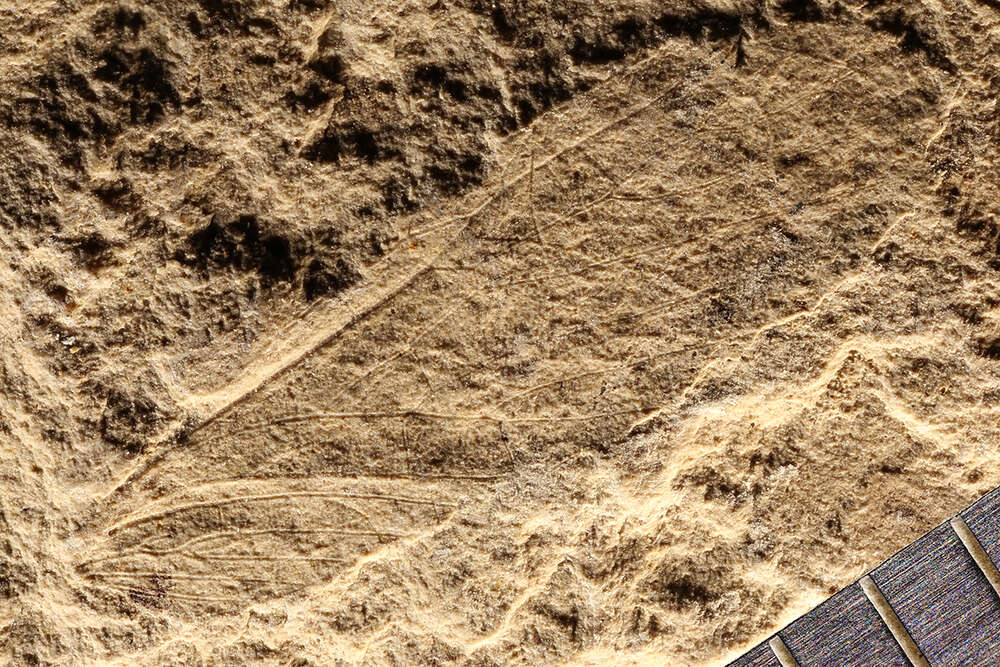The image depicts a primarily light brown, dry ground that resembles a mix of dirt and sand. It occupies most of the scene, with a fairly level surface concentrated on the middle and right-hand side, punctuated by vein-like cracks that resemble leaf patterns. The upper and left sections, however, appear patchier and slightly darker, as if the dirt has been disturbed or partially removed, creating an uneven texture. On the lower left corner, a fluffy, tannish-beige substance, possibly shredded wood or leaves, mimicking the appearance of sawdust or even fur in some clumps, covers part of the ground. Interwoven within this fluff are root-like structures branching out. In the lower right corner, there is a visible structure, potentially a roof or table, characterized by three distinct divider-like channels between its segments. The overall scene lacks a particular pattern but is marked by its earthy tones and varied textures.